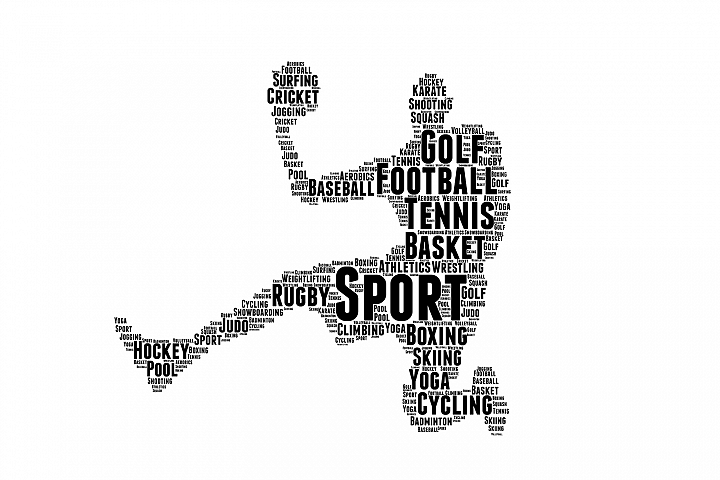The image features a dynamic, silhouette-like design of a basketball player, created entirely from a diverse collection of sports-related words arranged meticulously against a white background. The figure, positioned centrally, evokes an impression reminiscent of the iconic Michael Jordan 'Jumpman' logo, with the player captured mid-air, holding a basketball in one hand. The prominent words forming the athlete include "surfing," "cricket," "golf," "football," "tennis," "basket," "rugby," "boxing," "skiing," "yoga," and "cycling," while numerous other sports terms, such as "hockey," "karate," "shooting," "baseball," "athletics," "wrestling," "pool," "judo," and many more, intricately fill out the details. Rendered in stark black and white, the image suggests an artistic meme-like quality, designed for sharing across social media platforms.